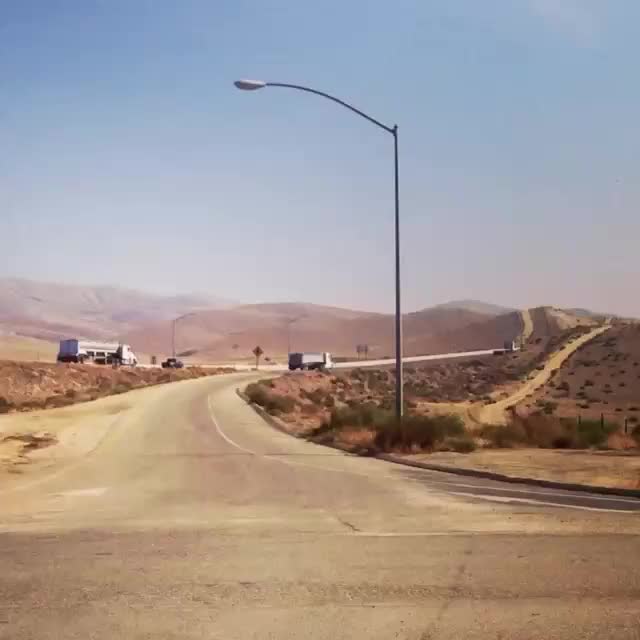This daytime color photo captures a desolate, run-down freeway stretching through a vast, mostly brown desert landscape with sparse green foliage. The main perspective is looking down the two-lane highway that seems to curve or intersect in the distance. Dominating the scene are small dirt hills and brown brush extending into the horizon under a bright blue sky. A prominent street lamp arches over the road near the foreground. On the freeway itself, two large trucks—a dump truck and a tanker-type truck—are seen driving, with the latter entering the highway. Additional features include faint road markings, subtle shadows, and a secondary driveway or street branching off to the right, all set against a backdrop of an indistinct mountain range.